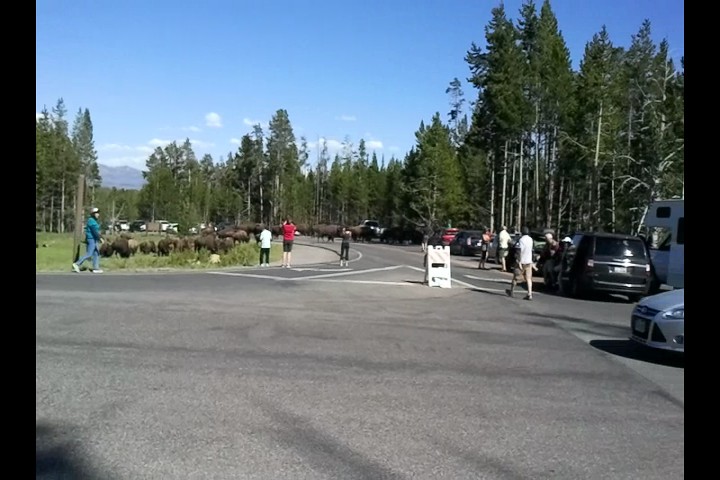The image depicts a scene in a dense forest area with a clear, blue sky decorated by a few clouds. The focal point is a large asphalt road where people are gathered, creating some form of event or activity centered around a herd of bison crossing from the left to the right side of the road. The road features a small white sandwich board, possibly serving as a caution or event sign, indicating restricted movement to accommodate the crossing animals. 

Numerous people, some wearing white t-shirts and shorts, are either guiding the bison or capturing the moment with their cameras. The scene involves a notable level of traffic, with vehicles, including an RV and two sedans (one black and one silver), lined up and halted to avoid hitting or disturbing the bison. The traffic congestion primarily occurs on the right side of the road, while a few passengers stand on the left, also taking pictures. The towering green-leafed trees form a dense backdrop, emphasizing the natural habitat and creating a picturesque yet bustling moment of coexistence between humans and wildlife.